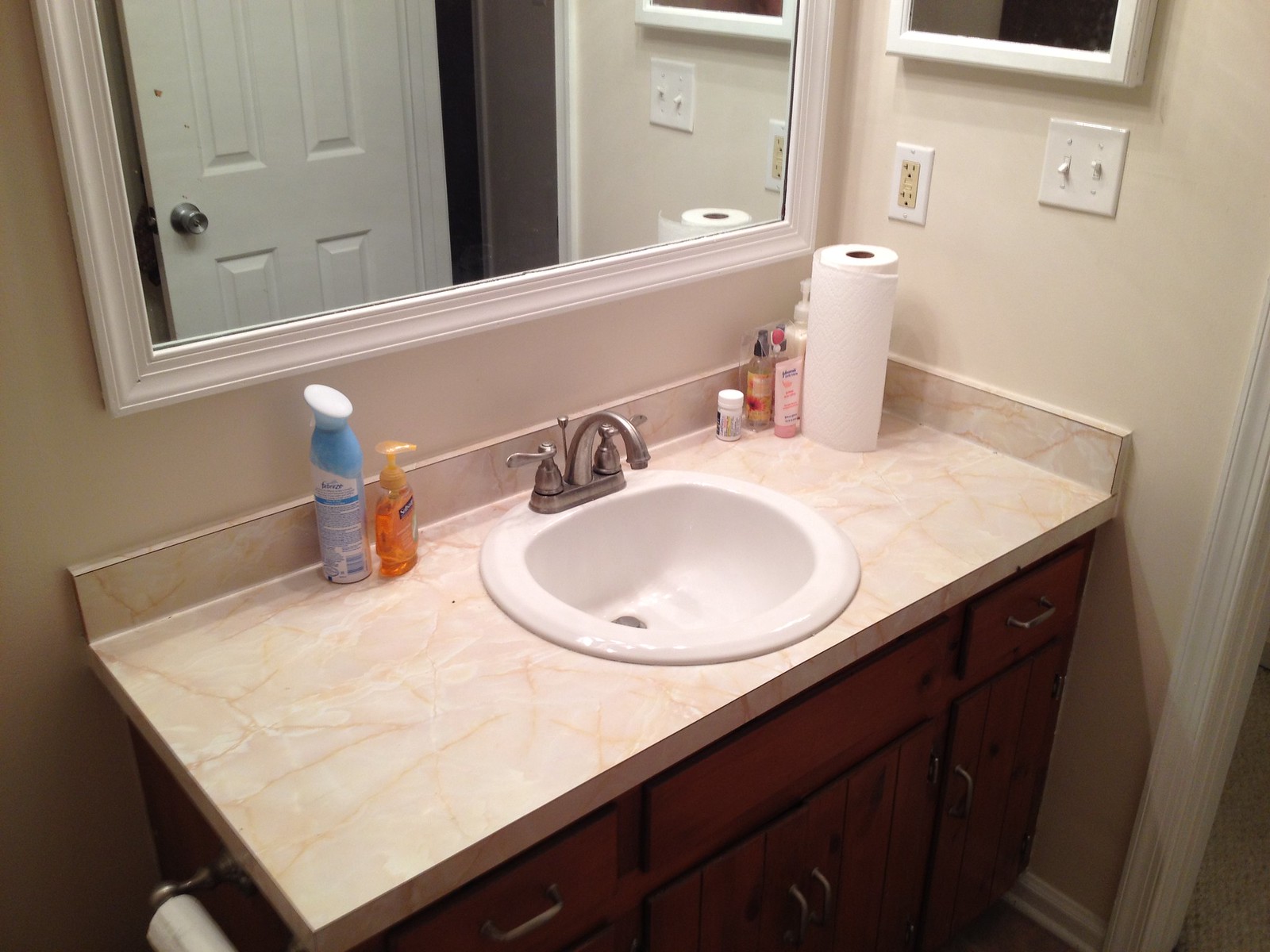This photo showcases a freshly renovated bathroom with a clean, modern aesthetic that you might see in a real estate listing on Zillow, or as shared by a friend who recently updated their home. The bathroom features a dual light switch and an electrical outlet installed on the wall. There is a framed photo partially visible, its lower edge peeking out from a white frame.

The doorway is accented with white trim, coordinating with the baseboards that line the floor. The sizable counter space is a blend of whitish and pinkish hues with subtle streaks, housing a single white sink. The faucet is a sleek chrome, adding a touch of modern elegance.

Dominating one wall is a large mirror framed in white trim that matches the doorway. The white door to the room sports a stylish gray handle. On the counter, there is an orange-colored Softsoap dispenser and a can of Febreze, though the scent is not discernible from the image. A roll of toilet paper is appropriately placed on the toilet paper holder.

In the far corner of the counter, there appears to be skincare products beside a roll of paper towels and what looks like a bottle of Advil, indicating thoughtful personal touches in this beautifully updated space.